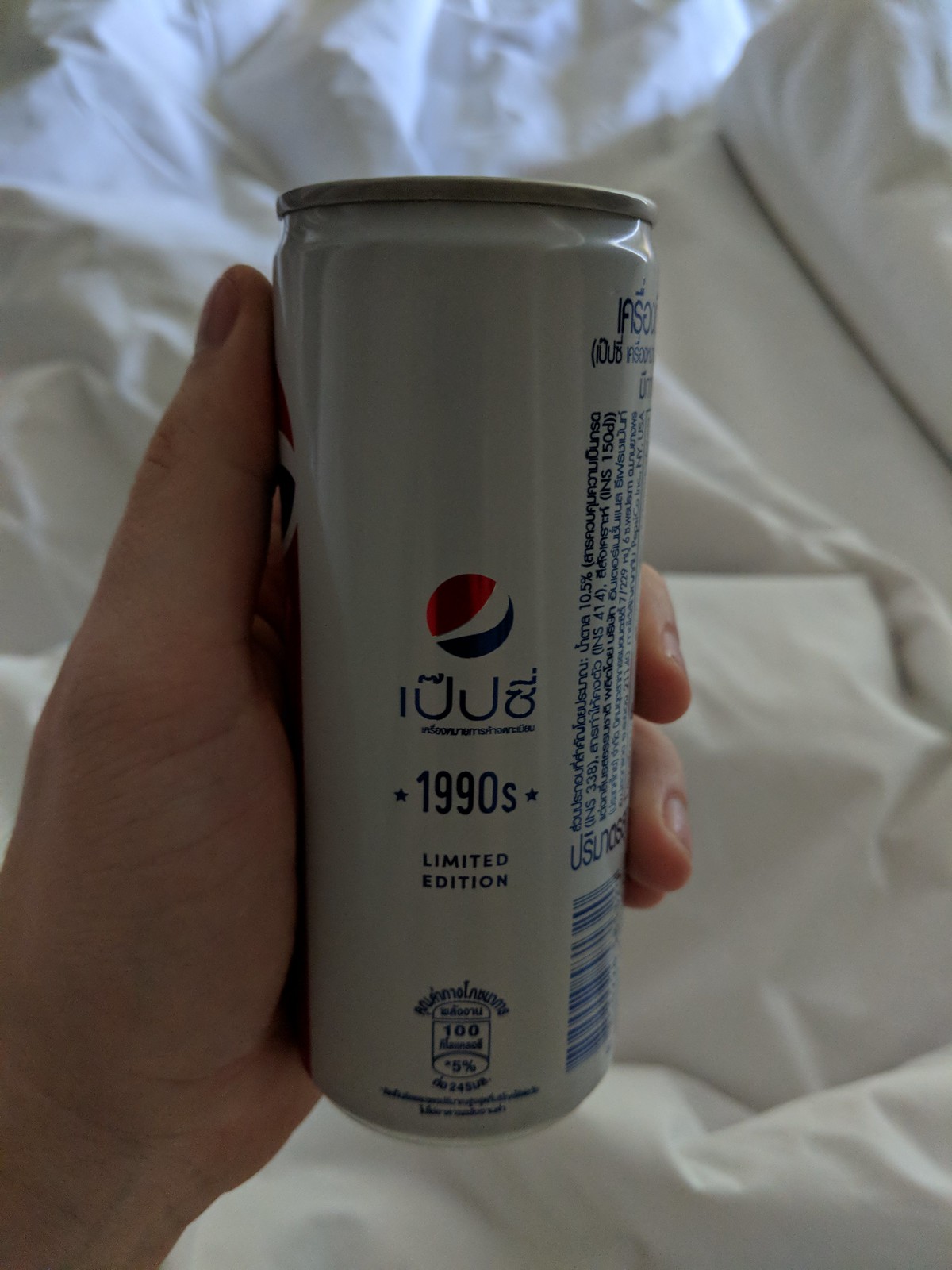A person is holding a white aluminum Pepsi can against a background featuring an unmade bed with white sheets and a pillow. The can is primarily white with a prominent Pepsi logo in the center, consisting of a red, white, and blue circular design. Below the logo, there are non-English letters, presumably Arabic, followed by the text "1990s" with a small star on each side, and below that, "limited edition" in blue. Near the bottom, there is another logo which includes the number 100. The right side of the can displays nutritional information in non-English letters and a blue-outlined barcode on a white background. The can is held in the left hand of the person, with their thumb and the tops of three fingers visible, displaying well-kept fingernails. The wrist and part of the thumb are also visible, providing a firm grip on the can.